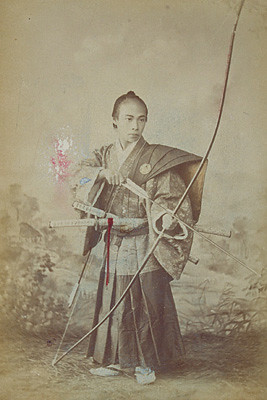The image is an old, sepia-toned photograph, likely from the mid to late 1800s, depicting a small yet imposing Japanese samurai warrior. The warrior stands at the center of the photograph against a painted backdrop of a field stretching into rolling hills. The sepia tones lend the photo a timeless, historical aura with shades of brown and beige dominating the image.

The samurai wears a traditional kimono with long sleeves and a pleated lower garment resembling a dress. The kimono features intricate patterns, possibly floral, spreading across the fabric. His feet are shod in white socks with sandals, reflecting the traditional attire of the era.

In his hands, the samurai clutches an extraordinarily long bow, nearly twice his height, indicative of its use for long-distance archery. His right arm is bent, holding the feathered end of a long arrow which stretches diagonally across the frame. At his waist, tucked into his sash, rest two sheathed swords, signifying his status and readiness for combat.

The warrior's hair is slicked back and tied in a topknot, displaying a high forehead. His facial expression is one of intense seriousness and unwavering focus. A slight splash of color is present, with a light pink spray near his elbow and a red ribbon wrapped around one of the sword sheaths, adding a subtle yet striking contrast to the overall monochrome palette of the image.